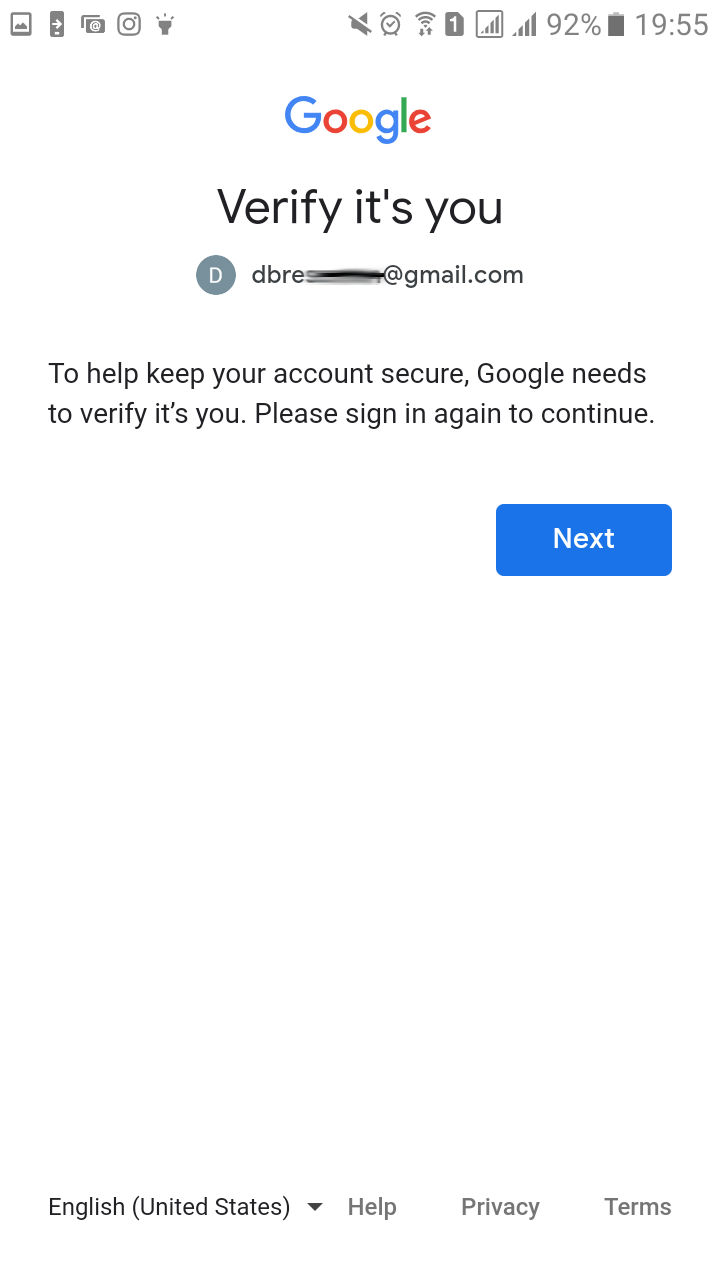This screenshot showcases the Google verification page on a mobile device. The top section features the Google logo centrally positioned. Directly below, bold text instructs the user to "Verify it's you." Beneath this heading, the user's Google profile photo is displayed, represented by the letter 'D'. Adjacent to the profile photo, to the right, is the user's email address, which has been obscured with a black mark for privacy. The message to the user reads: "To help keep your account secure, Google needs to verify it's you. Please sign in again to continue." Following this message, a prominent blue "Next" button invites the user to proceed to the next step. Additionally, the top of the screenshot displays various phone icons, including Instagram, the phone's photo gallery, sound, alarm, Wi-Fi, signal strength, battery percentage, and the current time.